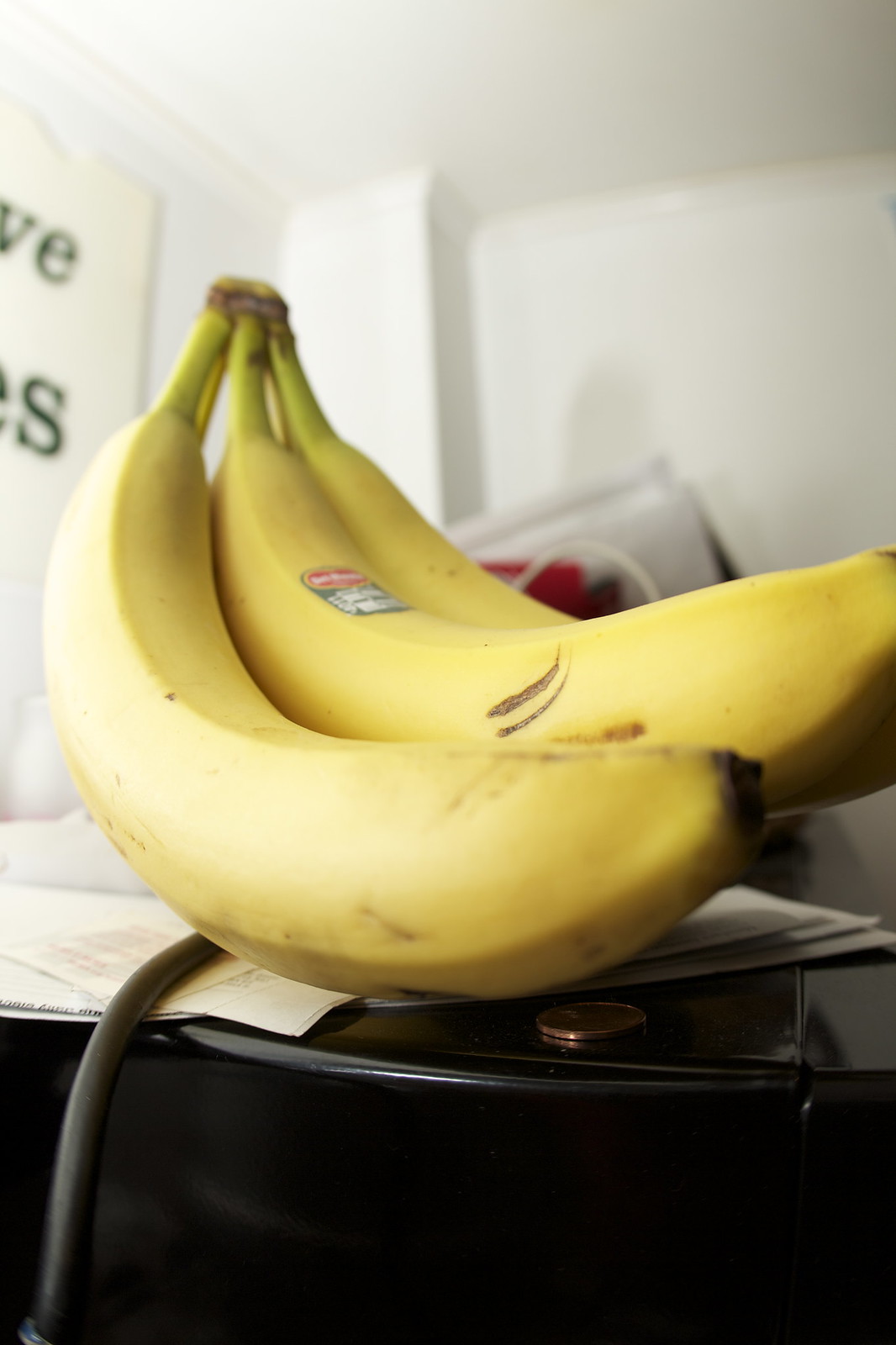A striking photograph features a cluster of bananas as its primary subject, prominently occupying the center of the image. The bananas are arranged on a glossy black surface, creating a stark contrast that highlights their bright yellow hue. Toward the left side, particularly in the upper left corner, the image captures partial text on the wall with the letters "V" prominently visible, followed by an "S" right below, suggesting a fragmented sign. 

In the immediate foreground beneath the bananas, a solitary penny lies on the black surface, adding a subtle detail to the composition. Scattered around the bananas are a few white envelopes or papers, contributing to the scene's everyday ambiance. From behind the bananas against the wall, there is a partially visible, blurry object that appears to be the corner of a square, gray item. Additionally, a small, indistinguishable red object towards the middle of the image adds a slight pop of color. This detailed setting captures the simplicity and commonplace nature of a moment centered around a bunch of bananas.